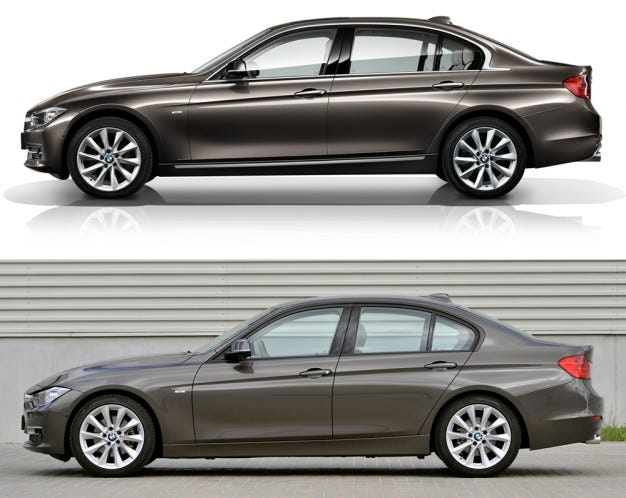This image displays two cars, one positioned above the other, highlighting a stark contrast between a glossy, ad-like portrayal and a more subdued, real-life setting. The top car is a sleek, metallic brown sedan with a shimmering, highly reflective surface, reminiscent of an advertisement. It features a gunmetal shine and a spacious, aerodynamic design that makes it appear new and stylish. The car's polished rims and clean, white backdrop enhance its visual appeal, giving it a sophisticated and modern look.

In contrast, the bottom car, which seems to be the same make and model, is presented in a more realistic context. Its brown color is noticeably duller, lacking the top car's vibrant sheen. Set against a background of horizontal tan-colored slats, likely the side of a building or garage, the car is parked on a concrete or asphalt surface. The rims on this car appear less attractive, contributing to its overall less polished appearance. The mundane grayish backdrop further diminishes its visual impact, making it feel more grounded and less striking than its top counterpart.